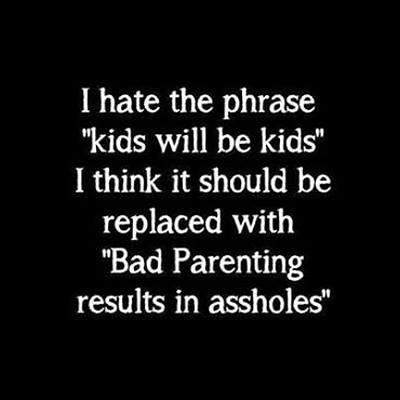This image features a prominently displayed quote against a stark black background. The square layout is completely filled with white text in a slightly worn, Times New Roman-style font. The quote reads: "I hate the phrase 'kids will be kids.' I think it should be replaced with 'bad parenting results in assholes.'" Notably, the phrase "bad parenting" is capitalized as "Bad Parenting." The simple yet bold design underscores the provocative message, with all text encased in quotation marks but lacking additional punctuation.